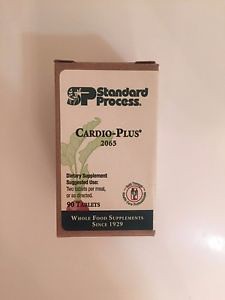The image portrays a vintage collectible rectangular cardboard box prominently displayed against a white background with a pinkish tint. The box shows signs of wear, with the flaps at the top being bent, indicating it has been opened and closed multiple times. The focal point of the box is the SP Standard Process logo, alongside the product name, "Cardio Plus 2065." This box contains a dietary supplement, specifically 90 tablets, emphasizing its health-related purpose.

On the front of the box, there's a subtle profile of a leaf, suggesting the health-oriented contents inside, potentially a whole food supplement, as indicated by the inscription "whole food supplements since 1929" at the bottom. The box also features an image resembling a root vegetable with accompanying green leaves, reinforcing the natural theme. The background consists of a soft, beige color mixed with off-white, enhancing the vintage aesthetic. A dark green stripe runs along the bottom of the label, bearing white letters which further detail the product description. The overall presentation of the box is of a well-worn yet distinguished health supplement item.